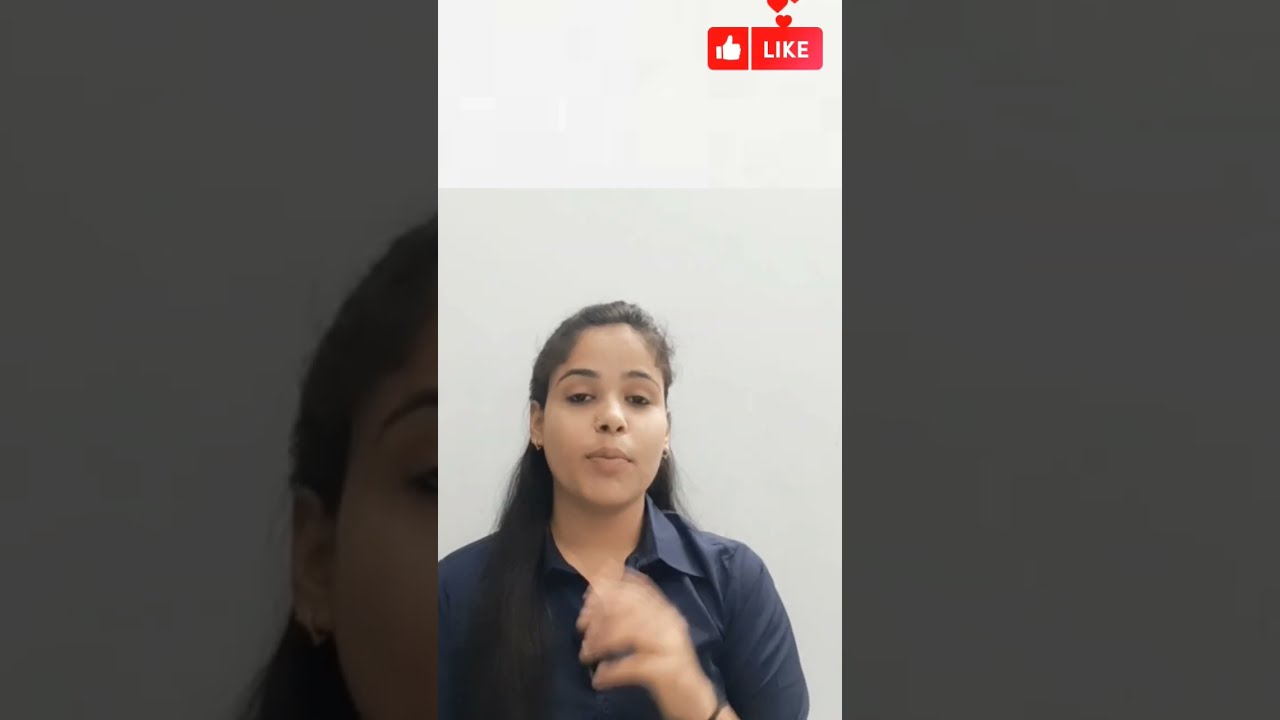The image is a horizontally aligned rectangular photograph divided into three vertical sections. The central section features a young woman, likely in her early 20s or 30s, with long black hair and cream-colored skin. She is wearing a dark blue collared button-down shirt and has small earrings. Her mouth is closed, and her eyes are looking directly at the camera, with her left hand slightly raised in front of her body, although it's a bit blurry. The background behind her is a gradient of gray, lighter at the top. 

In the upper right corner of the central section, there is a thumbs-up icon with the word "Like" in white against a red background, accompanied by several red heart shapes. The left and right sections of the image are close-up, darkened views of parts of the central photo; the left side shows an up-close view of the right side of her face, while the right side reveals a close-up of the wall in the background. The scene suggests she might be live-streaming or presenting in a video likely on a social media platform.